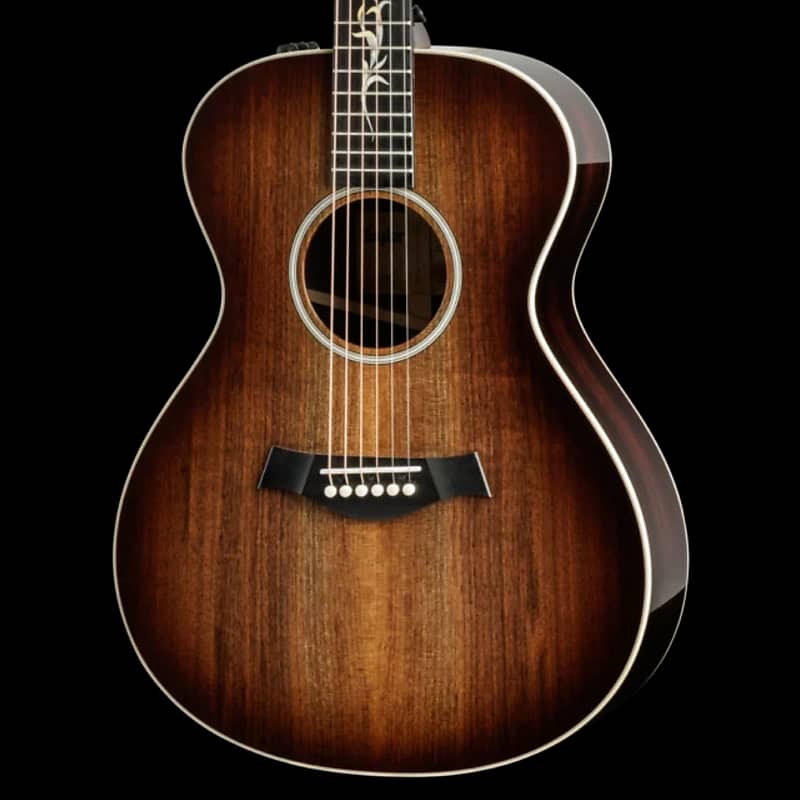A beautifully crafted guitar is showcased in the image, featuring a rich, dark brown finish that exudes elegance. The sides of the guitar glisten with a high-gloss sheen, enhancing the visual appeal of the vertical wood grain pattern that cascades down the instrument. The guitar's top part prominently displays a circular sound hole, encircled by a delicate white ring. This contrasts pleasingly with the dark wood. Below the sound hole lies a rectangular pickguard, protecting the guitar body, and alongside it, a set of pristine white strings stretches vertically down the guitar's length. Additionally, a sleek black plastic panel adds a touch of modernity and contrasts against the rich brown body. The guitar's sides feature a subtly wavy design, further accentuating its refined and sophisticated appearance.